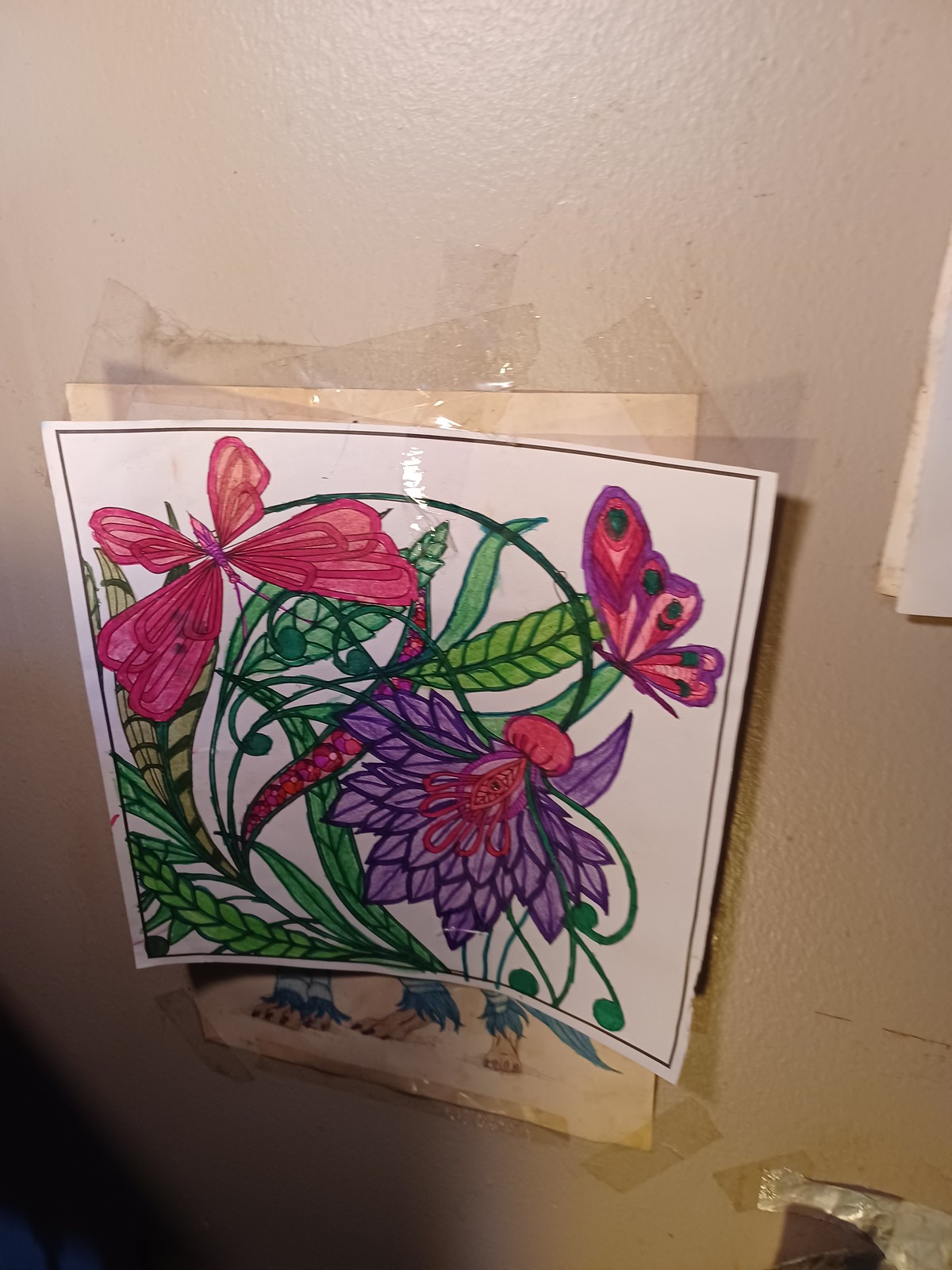The image depicts an intricate design created using markers on a piece of white paper, framed by a black border positioned just inside the edges. The central focus of the artwork is a large, vividly colored purple flower with a striking red center, surrounded by numerous green leaves in varying shades. Adding to the scene's charm, a butterfly with pink and purple wings adorned with blue and black spots hovers above the flower. On the other side, a larger butterfly with bold red wings illustrates the diversity of the scene.

The paper is affixed to a plaster wall painted in a light tan hue, using clear masking tape. The masking tape, appearing fresh, contrasts with the aged and dirty tape securing other pieces of paper visible on the periphery of the image. It's evident that this new artwork is taped over an older, partially obscured picture that remains on the wall. The juxtaposition of the new, vibrant marker drawing against the background of the timeworn elements adds depth and narrative to the visual presentation.